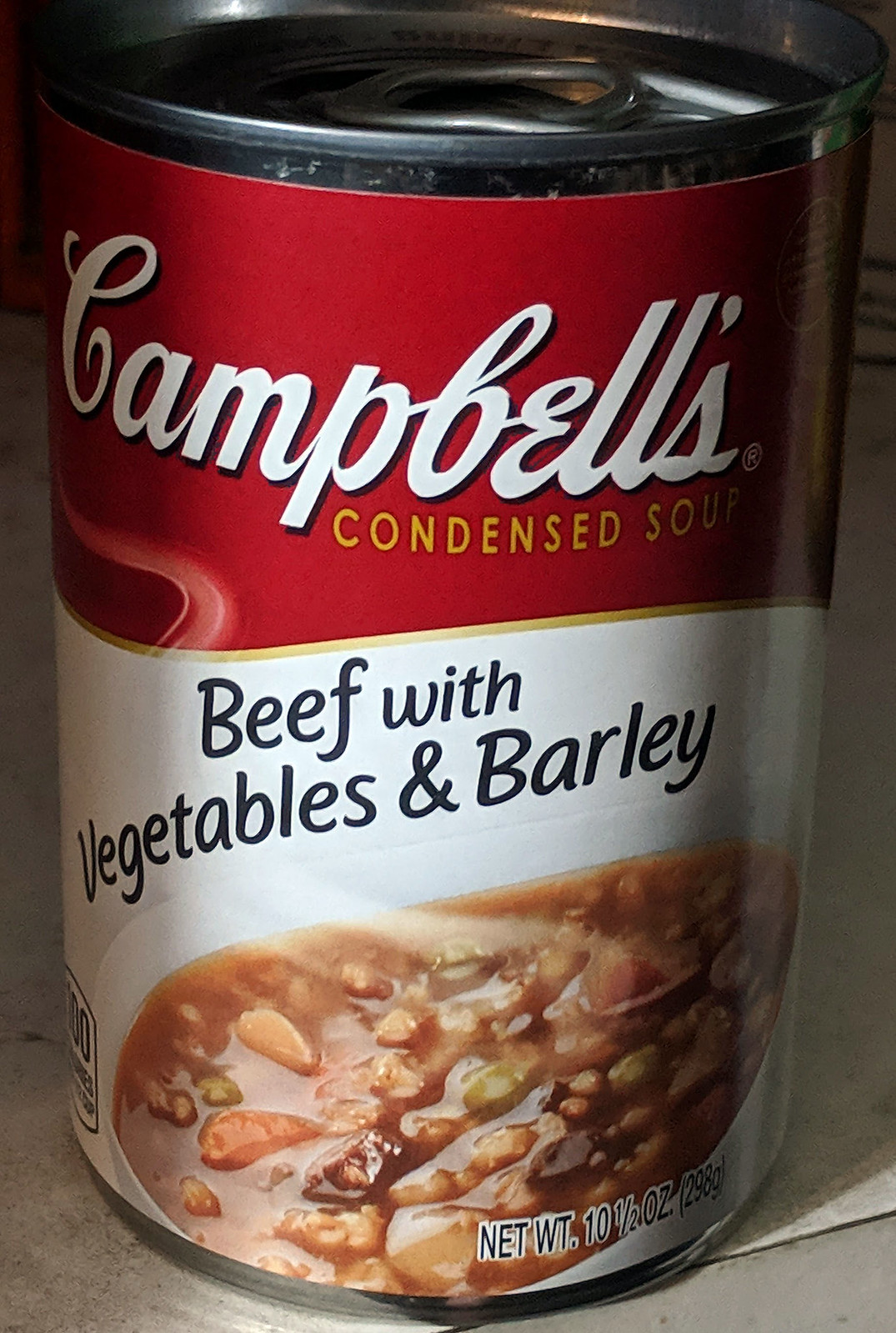This photograph is a close-up, portrait-mode image of a can of Campbell's Beef with Vegetables and Barley Condensed Soup. The can is silver with a pull-top tab, with the rounded part of the tab facing a bit to the right, and it sits on a worn and slightly dirty white Formica kitchen counter. The can itself features a red and white label. At the top, the iconic Campbell's logo is written in white cursive against the red background. Directly beneath that, "Condensed Soup" is displayed in bold yellow letters, still on the red background. A gold swirled line separates the red upper section from the white lower section. In this white area, it says "Beef with Vegetables and Barley" in black letters. A photograph of a white ceramic bowl filled with the soup occupies the lower section of the label, depicting brown broth with visible pieces of green vegetables, orange vegetables, and chunks of meat. At the very bottom of the label, in black letters outlined in white, the net weight is indicated as 10.5 ounces (298 grams). The can’s metal rim is slightly visible at the top, hinting that the label may have slipped a bit.